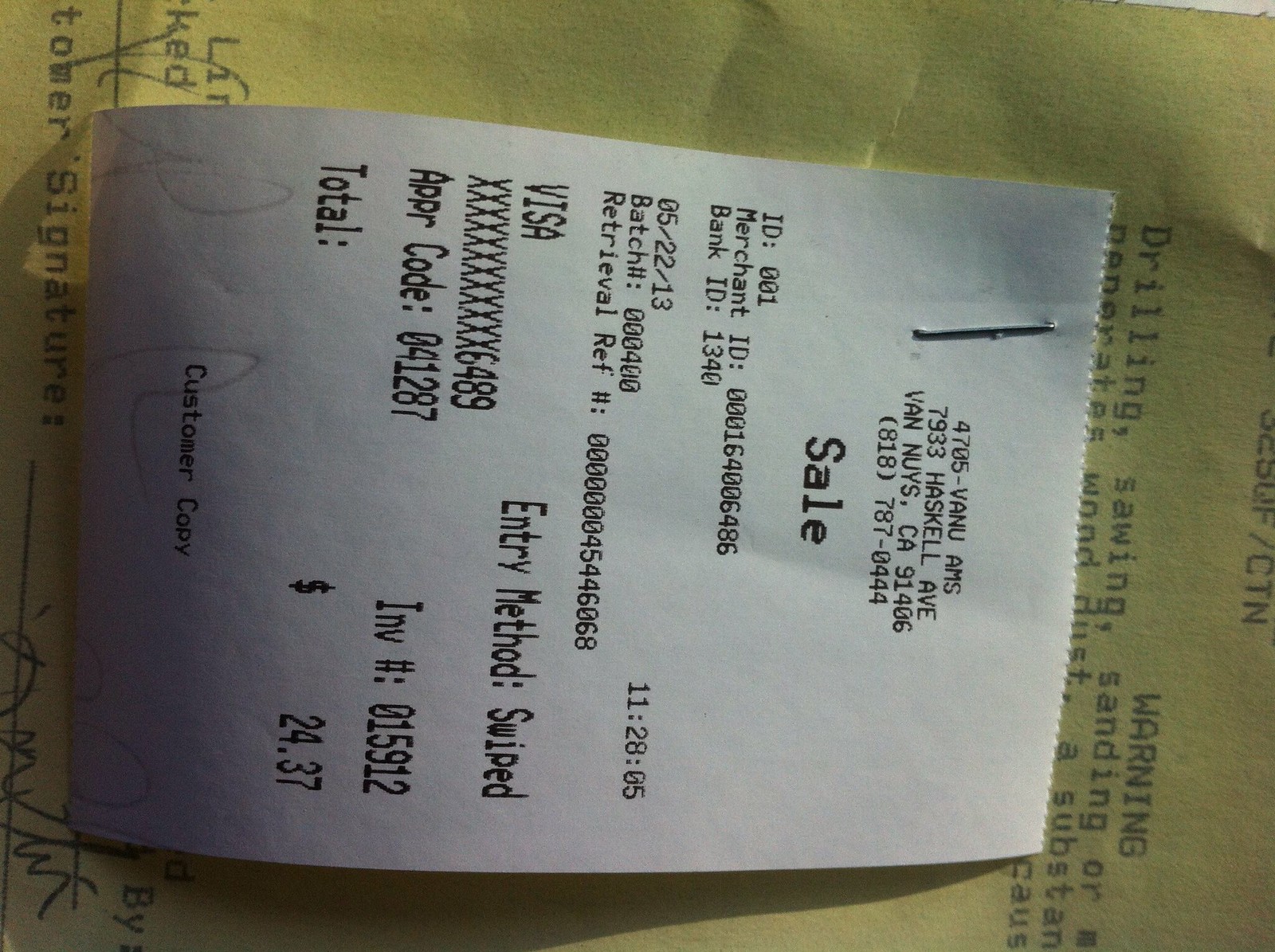The image is a close-up, landscape-oriented photograph, likely taken by a smartphone camera, of two receipts. A yellow receipt dominates the background, overlapped and stapled with a smaller white receipt in the foreground. Both receipts appear to be copies of the same transaction. 

The yellow receipt has partially visible text, including pre-printed safety information such as "CTN" and the phrases "drilling, sawing, sanding, or", followed by cut-off words further down. The background also displays a warning message that is not fully legible.

The white receipt, stapled on top of the yellow one, bears detailed information: the address "4705-VANU AMS, 7933 Haskell Avenue, Van Nuys, CA 91406 (818) 787-0444"; a bold "SALE"; and various transaction codes and numbers, including a merchant ID (0000164006486), bank ID (1340), and retrieval reference number (00000045446068). The receipt dates are displayed as "05/22/13" and "11-28-05". The payment method is identified by a Visa credit card, with a partially masked number ending in 6489 and an entry method labeled as "SWIPED". An approval code 041287 and an invoice number 015912 are present. The total amount of the transaction is $24.37. The bottom of the white receipt is captioned with "consumer copy, customer copy" and includes a signature line, although the signature is partially cut off in the image. 

Overall, the photograph captures the intricate details of a single retail transaction, with overlapping, stapled receipts providing multiple layers of information.